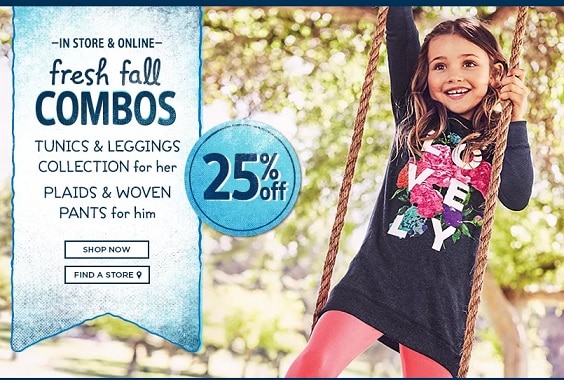**Descriptive Caption:**

A vivid, eye-catching advertisement for fall fashion, showcasing a delightful collection for all. The ad is dominated by a large, prominent "25% OFF" written in the largest font on the display, enclosed within a bold blue circle, immediately drawing attention. The text "In Store and Online," "Fresh Fall Combos," "Tunics and Leggings Collection for Her," and "Plaids and Woven Pants for Him" are creatively spread across the banner, appearing as if they are hanging from the top of the page, slightly swaying. Just below this lively text display, two blue-button options, "Shop Now" and "Find a Store," are neatly placed to prompt action.

Adding a touch of charm and warmth to the ad, a photograph of a joyful young girl, possibly around four or five years old, graces the background. She has long, dirty blonde hair and exudes a contagious smile as she stands on a swing, gazing happily to the left of the camera. Her presence on a swing adds a playful, whimsical touch to the advertisement, perfectly complementing the fresh and vibrant fall marketing campaign.